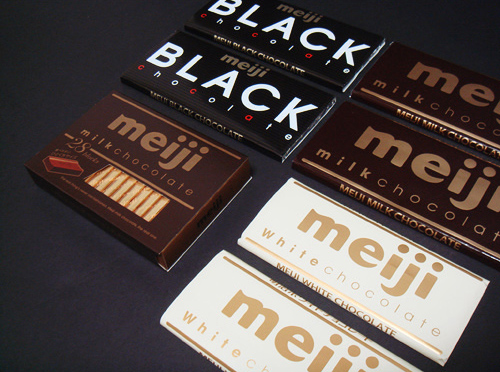This image features an array of seven Meiji chocolate bars arranged on a black surface. In the lower right corner, there are four bars aligned in a row, all branded with the name "Meiji" prominently printed in gold. The two lower bars in this row have white packaging labeled as "Meiji White Chocolate," while the two upper bars have brown packaging, indicating "Meiji Milk Chocolate." To the left of this group is another row of three chocolate bars. At the bottom of this row is a brown-wrapped "Meiji Milk Chocolate" bar with light brown lettering. Above this, there are two bars in black packaging with bold white lettering, labeled "Meiji Black Chocolate." The detailed image showcases the variety of Meiji chocolate offerings, highlighting the distinctions between their black, milk, and white chocolate flavors against the stark black background.